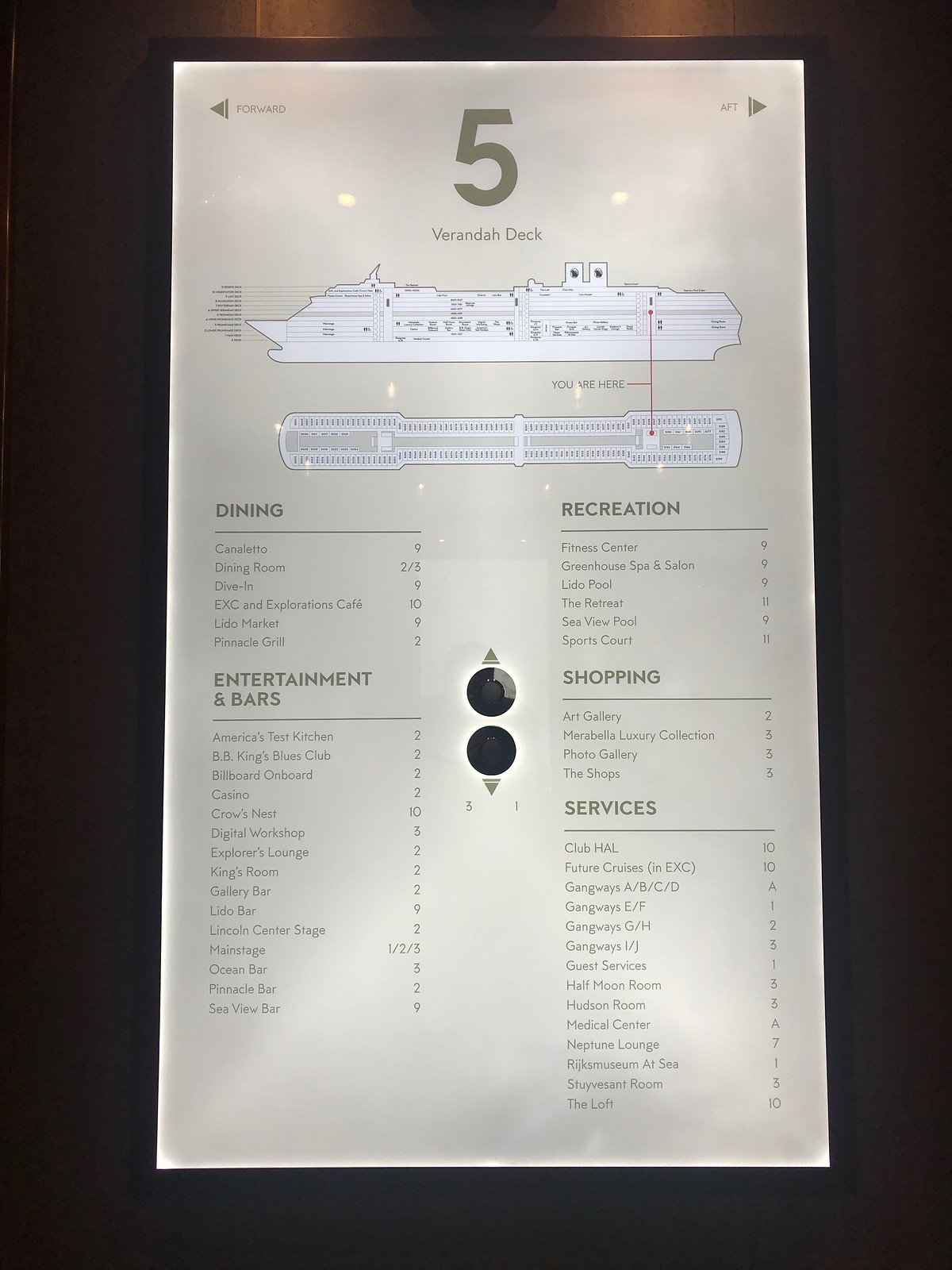This image features a detailed poster likely found on a cruise ship, prominently displaying information to help passengers navigate various amenities. The poster is set against a wooden background, with the sign itself being white and the text in dark gray or black. At the top of the sign, the number "5" is highlighted, indicating the viewer is on level five, often referred to as the "Veranda Deck" in light gray lettering just below the number. 

The center of the poster showcases a black sketch outline of the ship in a cross-sectional view, portraying its internal layout as if the vessel has been sliced in half. This side profile includes several labeled lines denoting different decks and categories. Specific categories such as dining, entertainment, bars, recreation, shopping, and services are detailed, showing what can be found on each level of the ship. Additionally, a vertical red line runs down the poster, marking the current floor and helping with orientation. Each category lists particular venues or facilities available, providing a comprehensive guide for passengers to find their way and discover various offerings on the cruise ship.